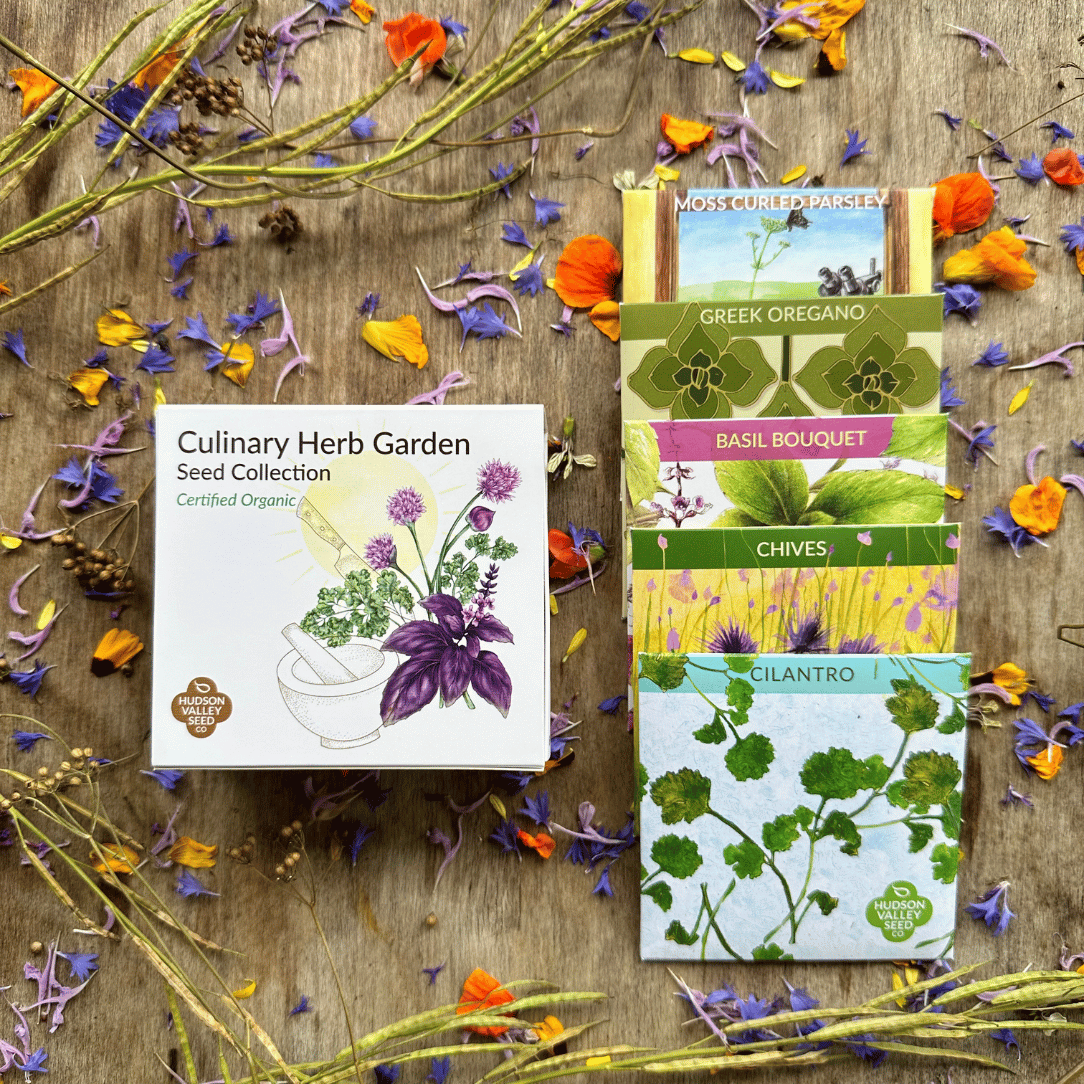This image is a detailed advertisement for a certified organic Culinary Herb Garden Seed Collection from Hudson Valley Seed Co. The color indoor photograph is taken from above, capturing a rustic wooden table with a prominent, textured medium-brown grain. On the left side of the table is a white packet with green lettering that reads "Culinary Herb Garden Seed Collection." Below that, it says "Certified Organic" and features a watercolor painting of a mortar and pestle along with various herbs and a purple flower. On the right side, there is a neatly stacked collection of seed packets, each adorned with watercolor illustrations of their respective plants. The visible packets from top to bottom include "Moss Curled Parsley," "Greek Oregano," "Basil Bouquet," "Chives," and "Cilantro." Surrounding the packets are scattered, dried florals in hues of purple, yellow, and orange, along with twigs and sticks, adding a decorative touch to the rustic presentation.